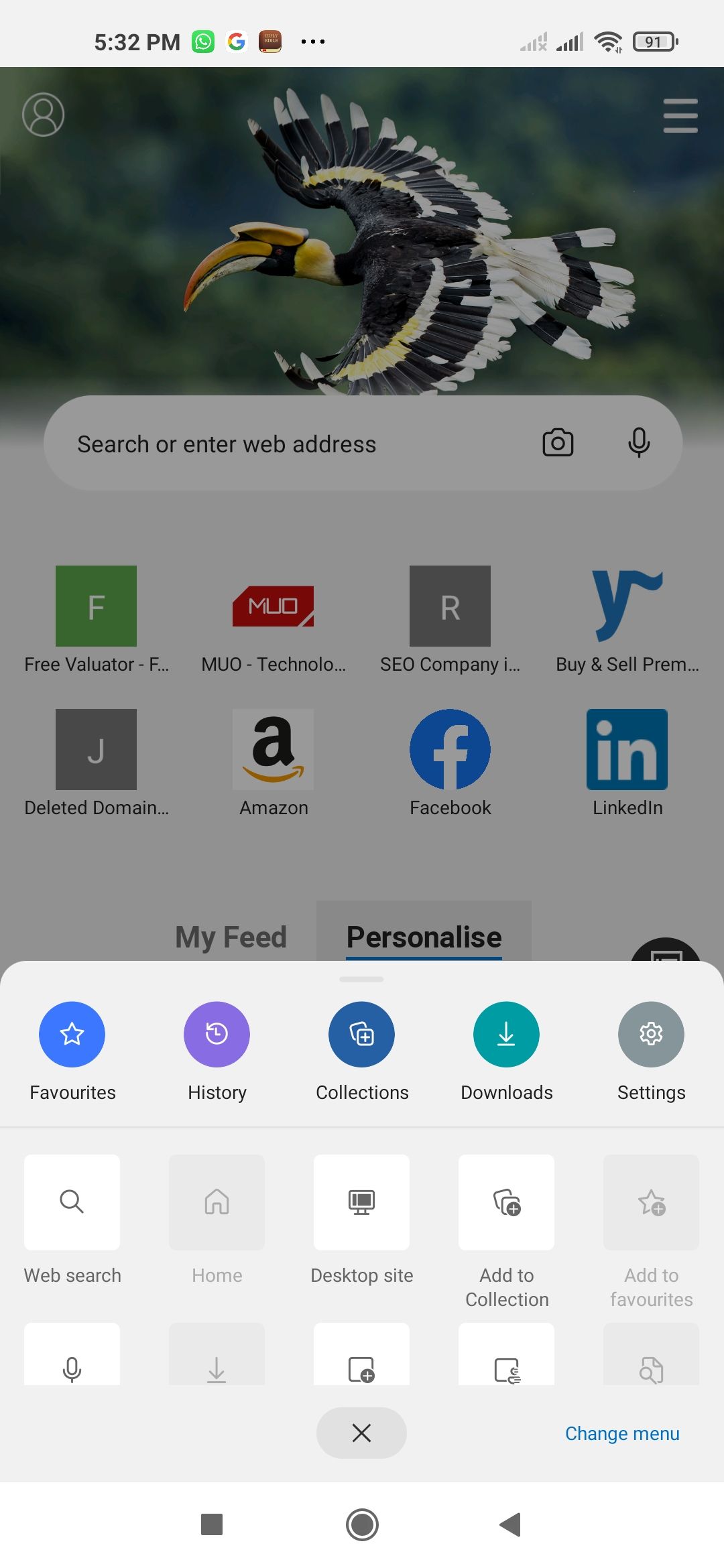In this detailed screenshot of the Nubar device, the image prominently features the device's interface. At the very top, the status bar displays key information: the time is 5:32 p.m. located in the top left corner. Various notification icons are visible, including those for WhatsApp, Google, and the Holy Bible. To the right, there are two network signal bars; SIM 1 indicates 'No SIM,' while SIM 2 shows a strong signal with 4 out of 5 bars. The Wi-Fi connection is at full strength, displayed with 4 out of 4 bars. Additionally, the battery level indicator reads 91% charged.

The primary focus of the image appears to be a web page, but the specific content of the page is not clearly described in this context. The home screen apps visible on the Nubar device are diverse, including Free Valuator, Amazon, Facebook, LinkedIn, SEO Company, Buy and Sell, My Feed, Personalize, Travel Rights, and History. Each app icon is distinctly displayed, suggesting a well-organized and user-friendly interface for easy access to various services and functionalities.